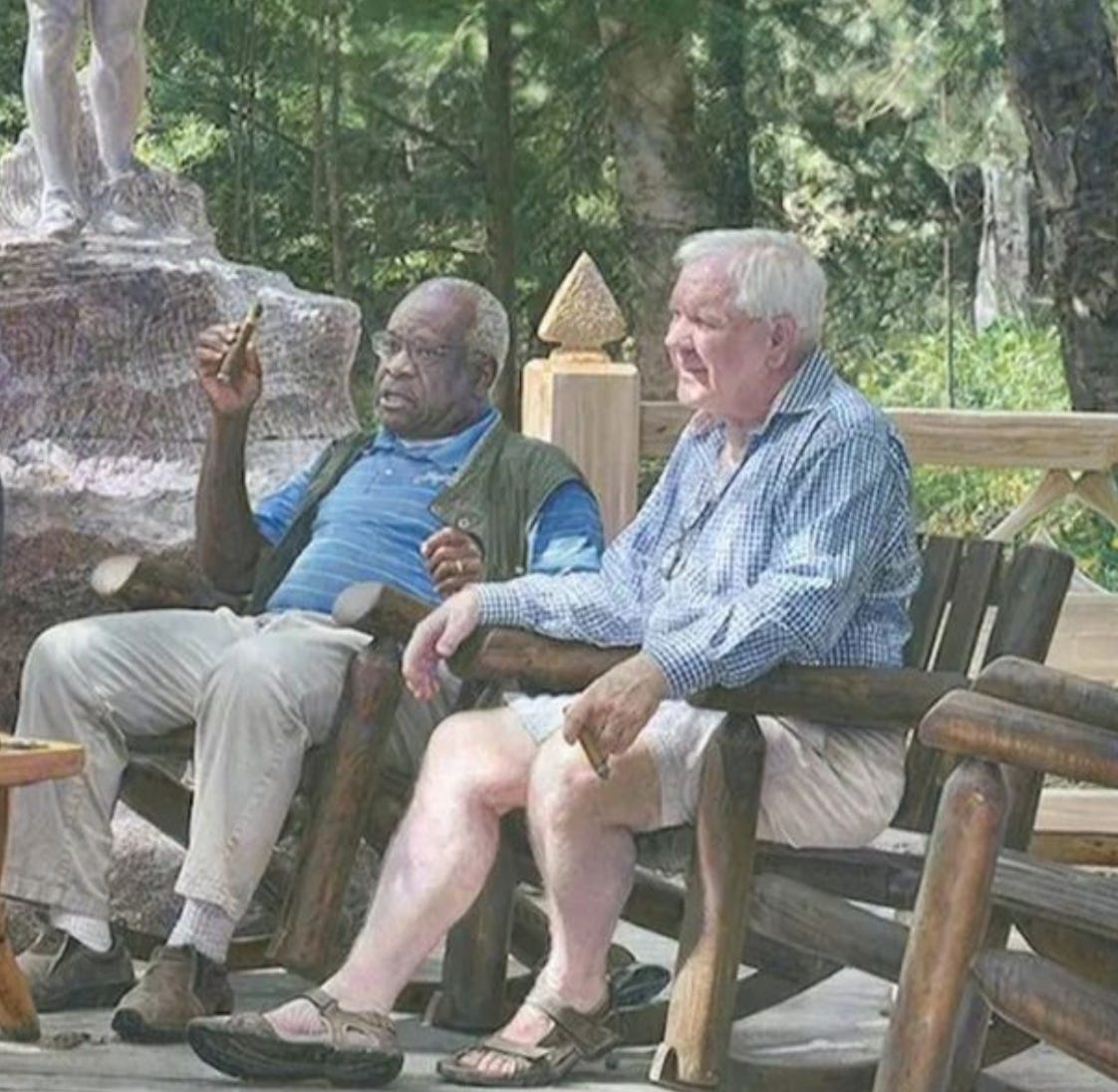The image features two older gentlemen seated in rustic, log-style wooden rocking chairs, facing the left side of the frame. The man on the far side, an African-American with short gray hair, is dressed in a blue polo shirt with white stripes, a green vest, khaki pants, and brown slip-on shoes. He is smoking a cigar with his right hand. Beside him sits an older white man with white hair and glasses hanging between the buttons of his blue and white plaid long-sleeved shirt. He wears khaki shorts, brown sandals, and holds a cigar in his left hand. Behind them is a light tan wooden fence, partially obscuring a stone statue visible at its base, with a forested area extending into the background. The image appears somewhat faded, suggesting it could be an aged photograph. Despite the peaceful setting, there's an uncanny feeling about the image.